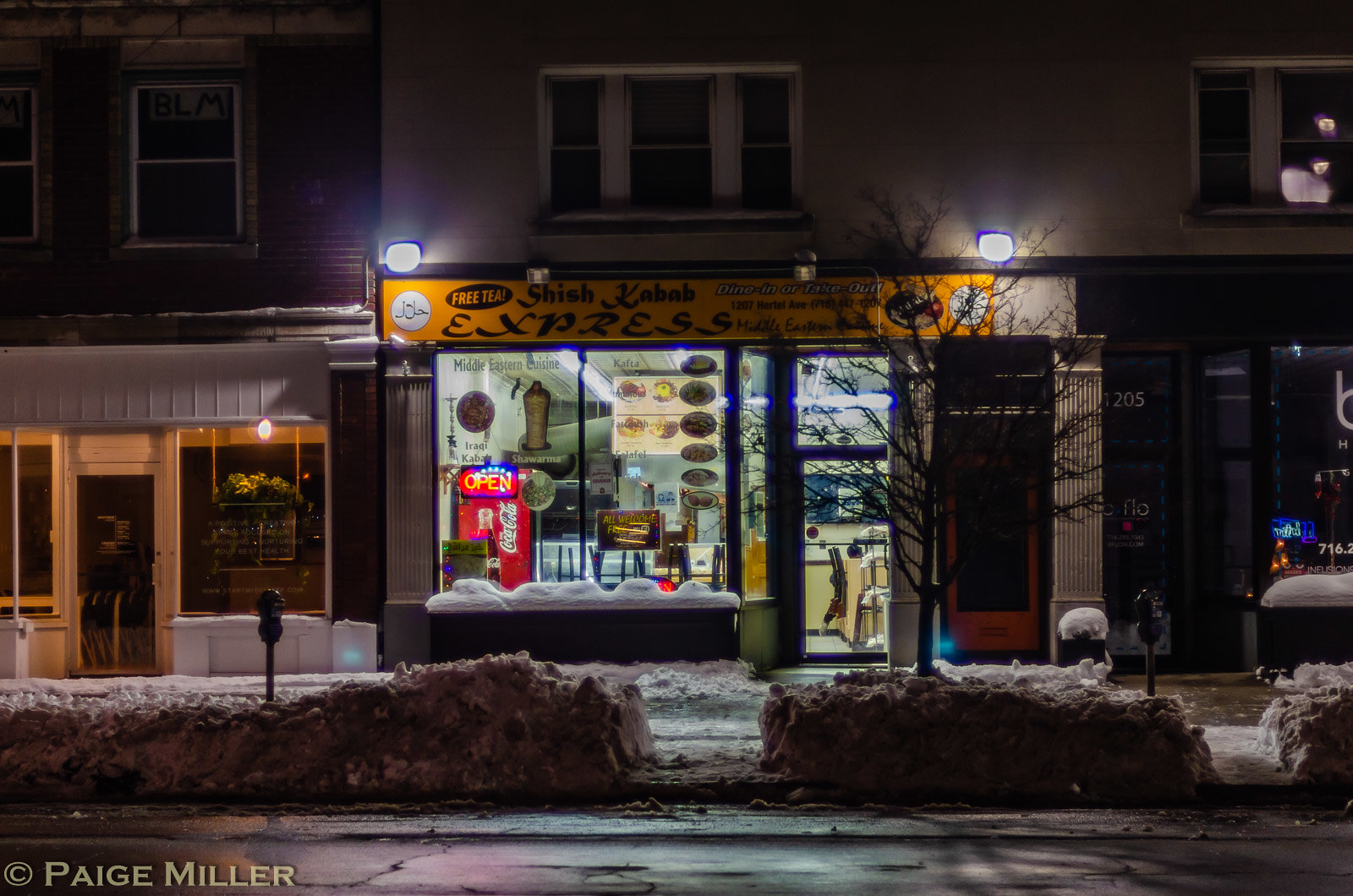This photograph, taken at night by Page Miller, captures a snowy street scene focusing on a row of stores with a particular emphasis on a brightly lit shish kebab restaurant in the center. The image, rectangular and wider than it is tall, showcases a serene winter night where thick snow blankets the sidewalks and median, partially covering parking meter poles and a tree trunk, and forming pathways cleared through the snow. In the middle of the frame, the shish kebab restaurant stands out with its lights on and an illuminated "Open" sign visible through the large glass windows and doors, which provide a glimpse inside to empty chairs turned upside down on tables and a Coca-Cola machine. Above the entrance, a yellow banner with black text reads "Free Tea Shish Kebab Express, Dine In or Take Out," with additional unreadable text. The stores adjacent to it are closed, enhancing the inviting glow of the open eatery amidst the quiet, snowy night.